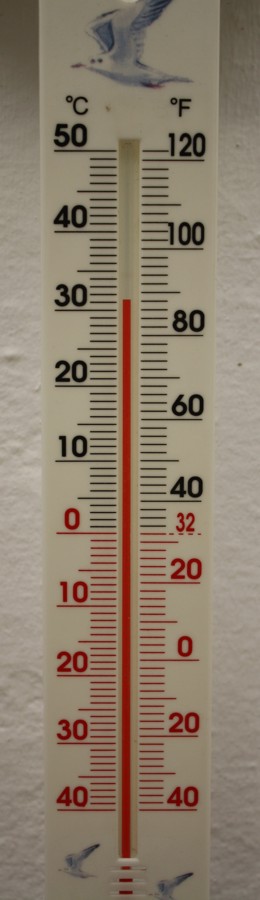This is a detailed top-down photograph of a plain white thermometer. The thermometer, which could be either mounted on a wall or lying flat on a table, displays temperatures in both Celsius and Fahrenheit. The Celsius scale is located on the left with red text for sub-zero temperatures: 40, 30, 20, 10, and 0, and black text for positive temperatures: 10, 20, 30, 40, and 50. On the right side, the Fahrenheit scale starts from the bottom with red text numbers: 40, 20, 0, 20, and 32, followed by black text numbers 40, 60, 80, 100, and ultimately 120 at the top of the scale.

Artistically incorporated into the thermometer's design are three flying birds. At the bottom of the thermometer, there are two smaller birds in mid-flight. Higher up, at the top of the thermometer, there is a slightly larger bird that closely resembles a seagull, providing a simple yet charming touch to the functional design.